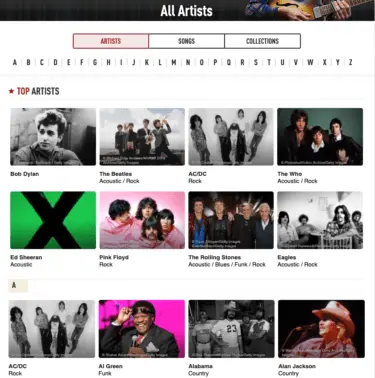This image is a rectangular screenshot of a music website, showcasing its "All Artists" section. At the top, there is a black rectangular banner with white text that reads "All Artists," positioned beside a photograph of a person holding a guitar or bass. Below the banner are three clickable buttons, indicating different sections of the site. The first button, labeled "Artists," is currently selected, highlighted with a red border, light red background, and red text. 

Adjacent to the "Artists" button are two additional buttons: "Songs" with a white background and black border, and "Collections" on the rightmost end. The background of the website is predominantly white. Beneath the "Top Artists" header, which features "Top" in red text and "Artists" in black, there is a display of top artists, likely sorted alphabetically. This section is further facilitated by an alphabetical list, where each letter is individually clickable.

The main display area showcases three rows, each containing four rectangular images representing various artists. Alongside each image is likely the artist's name and genre. For example, on the leftmost position of the first row is Bob Dylan, and in the lower right corner under the letter "A" section is Alan Jackson, a renowned country musician. Below each artist's name, their respective music genre is typically indicated.